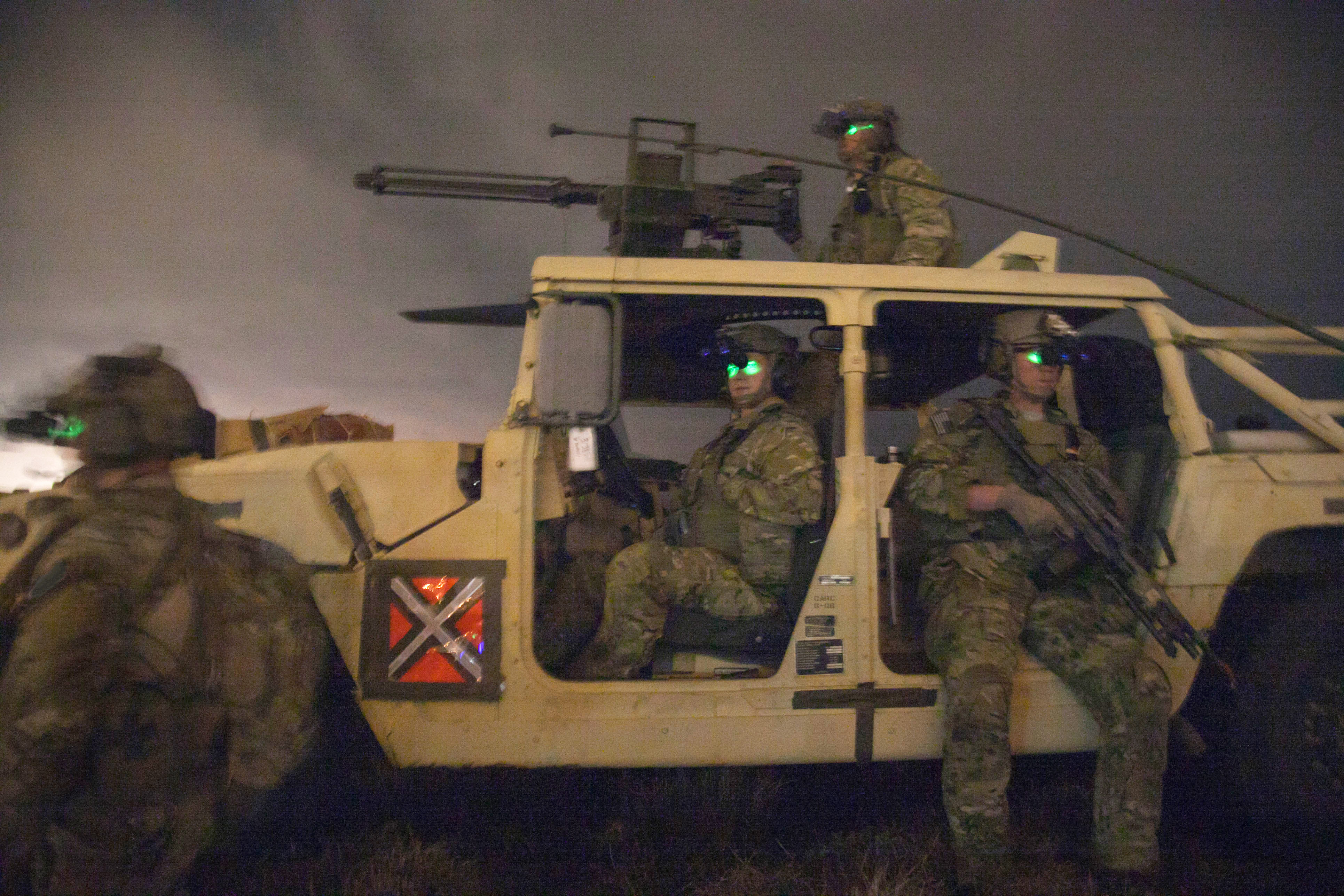In this detailed photograph set against a tan background, a tan Desert Storm military Humvee is depicted amidst smoky or cloudy dusk skies, suggesting a nighttime or evening operation. The vehicle, devoid of doors, houses three U.S. soldiers sporting desert camouflage fatigues, olive and tan helmets, and night vision goggles that cast a distinctive green glow on their eyes. The soldier in the driver’s seat is ready to maneuver the vehicle, while another in the rear seat has his legs dangling out, a machine gun resting across his chest. Atop the Humvee, a fourth soldier, similarly attired, stands behind a mounted large machine gun pointing towards the left, prepared for action. A red square patch bordered in brown with a white cross is taped or affixed to the left front quarter panel of the Humvee. Outside the vehicle, near the front left, stands another camo-clad soldier, viewed from the back, adding to the intensity and readiness captured in this scene.